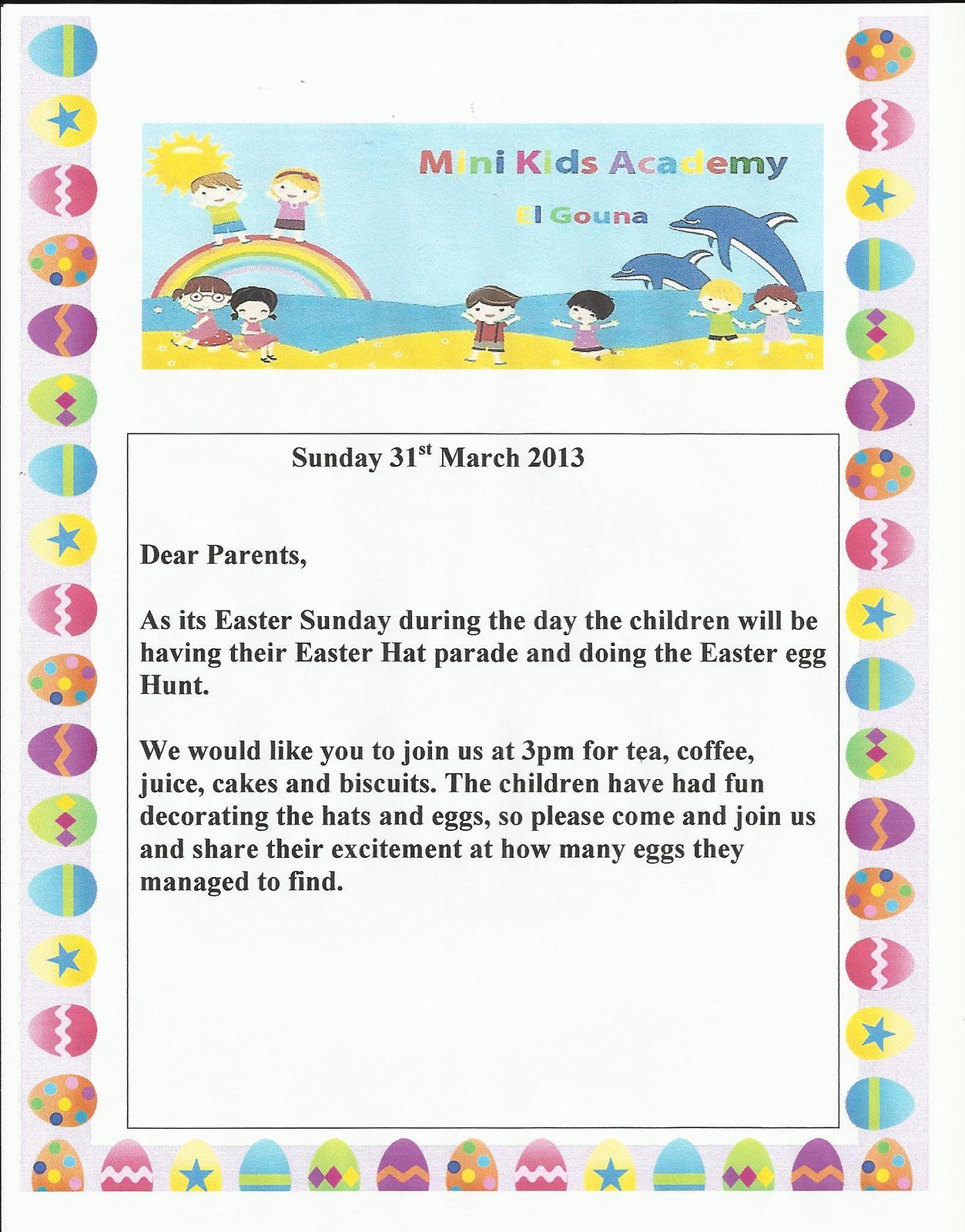The image is a scan of a piece of paper from Mini Kids Academy dated Sunday, 31st March 2014, inviting parents to an Easter event. The letter, set on a white backdrop with black text, reads: "Dear Parents, as it's Easter Sunday, the children will be having their Easter hat parade and doing the Easter egg hunt. We would like you to join us at 3 pm for tea, coffee, juice, cakes, and biscuits. The children have had fun decorating hats with eggs, so please come in and join us and share the excitement of how many eggs they managed to find."

The border of the paper is adorned with colorful illustrations of Easter eggs on a light blue patterned background. Among the designs, there's a yellow egg with a blue star in the middle, a blue egg with a yellow band, and a yellow egg with diamonds of various colors around the middle. At the top of the letter, a vibrant scene features children playing in a grassy field, a rainbow, and blue dolphins leaping through the air. The setting is cheerful and outdoorsy, rendered in a playful cartoon style, capturing the festive spirit of Easter and the joy of children's activities.